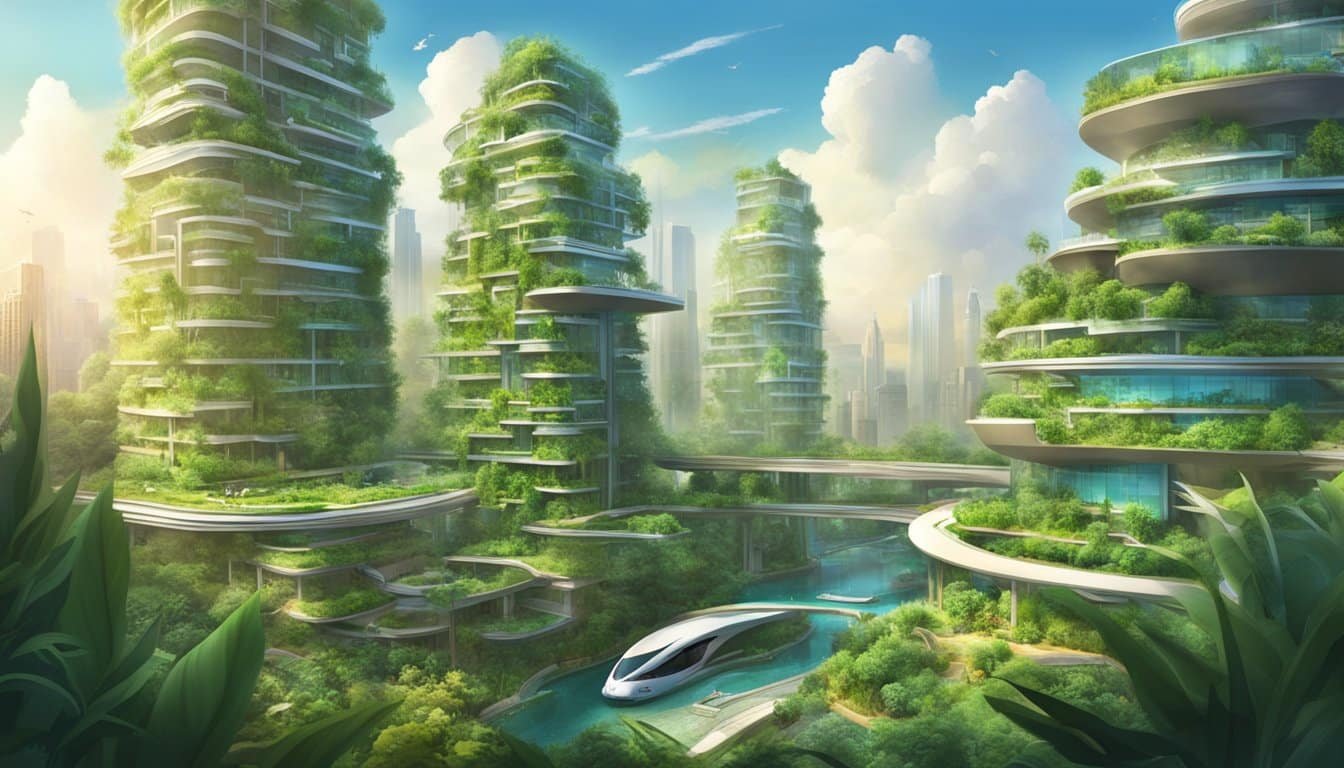This highly detailed, horizontally aligned, digitally created image portrays a futuristic utopian scene reminiscent of a video game landscape. The backdrop features a bright sky with large, puffy cumulus clouds, and some thin, feather-like ones in the middle. In the upper left, transitioning towards the center, there are towering rectangular buildings, distinguished by multiple levels adorned with abundant greenery, including grass and trees on balconies and rooftops. A unique circular building on the right spirals to a narrow top. The foreground displays large leaves in both the lower left and right corners.

Centrally, a narrow, light blue canal hosts a modern water vehicle resembling a metro train. This sleek shuttle-like boat, white with black windows, traverses the canal. The scene also includes interconnected highways and bridges adorned with grass, trees, and bushes, enhancing the utopian essence of the artwork. The image, devoid of a signature, combines elements of futuristic architecture and lush greenery seamlessly, exemplifying a harmonious blend of technology and nature.